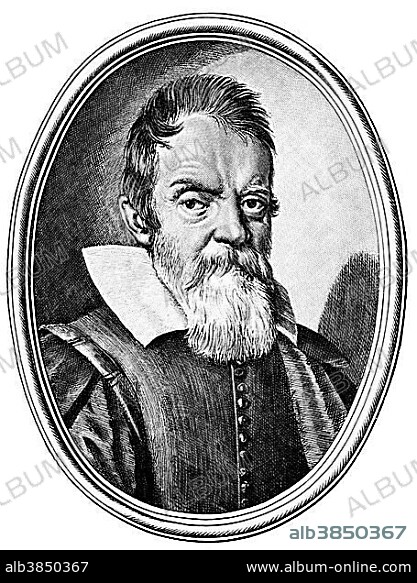This detailed, black and white hand-drawn illustration, likely depicting Galileo, features a bearded man in early modern garb, appearing to be in his late 50s or 60s. Framed in an oval hand-drawn border, the subject has medium-length hair brushed to the side and a long, gray beard with a matching mustache, complementing his serious expression and wide eyes. He wears a distinctive outfit comprising a large white collar, a button-down single-breasted shirt, and puffy sleeves. Watermarks span across the image, including "album" prominently displayed, with the notation "ALB3850367 www.album-online.com" at the bottom.